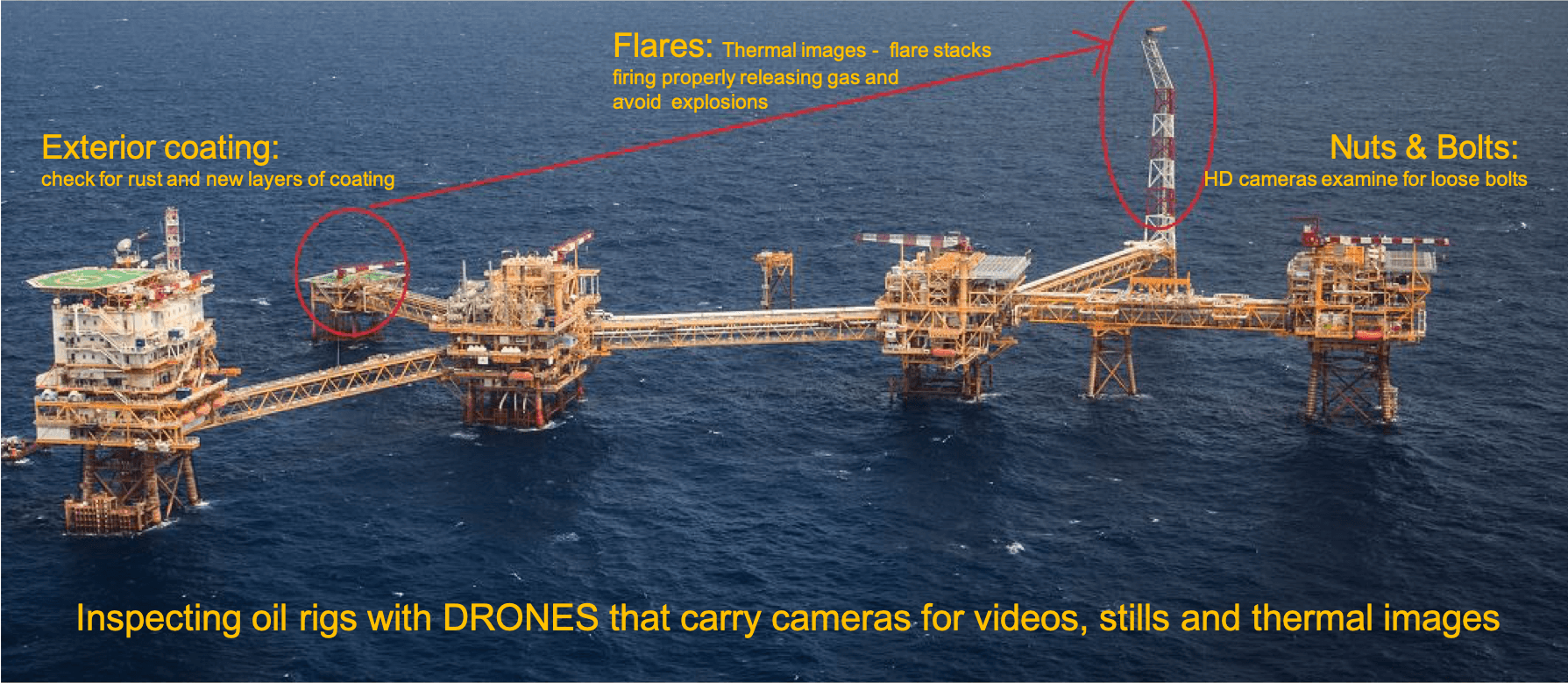The image depicts a series of interconnected oil rigs, with vibrant orange and white metallic structures set against the calm waters of the ocean, captured in a realistic and detailed aerial photograph. In the center, multiple rigs are connected by bridges, and a helicopter pad is clearly visible atop one of the sections. The photograph features overlaid text and annotations, spotlighting various inspection details. Prominent yellow text at the bottom reads: "Inspecting oil rigs with drones that carry cameras for videos, stills, and thermal images." Additional annotations include guidance for various components: on the left, "Exterior Coating: Check for rust and new layers of coating"; at the top, "Flares: Thermal images; flare stacks firing properly, releasing gas, and avoiding explosions"; and on the right, "Nuts and Bolts: HD cameras examine for loose bolts," with corresponding arrows and circles for visual emphasis.